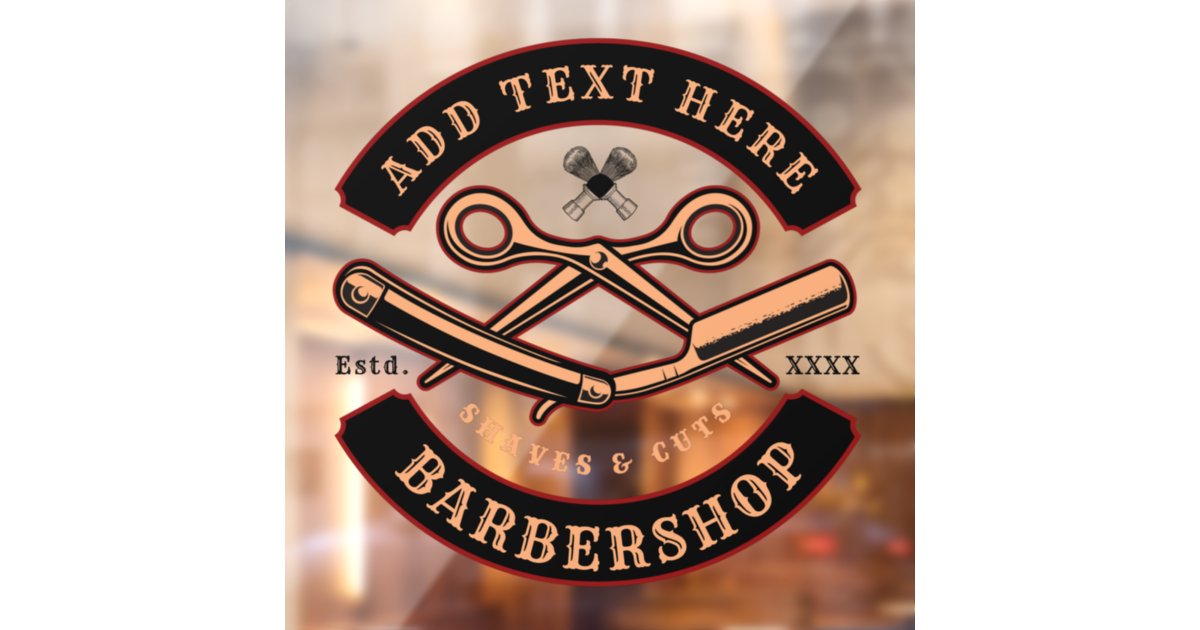This image showcases a customizable logo template for a barbershop, designed with a modern, contemporary feel. The square logo features two thin and narrow semicircular banners. The top banner is designated for the name of your barbershop with the placeholder text "Add Text Here," while the bottom banner reads "Barbershop." The design is primarily in black and gold, accented with muted background shades of reds and different browns, creating a bright and eye-catching appearance.

At the center of the logo, there are vintage-style graphics including an open pair of scissors and a straight razor, both rendered in light gold or copper tones. The text "shaves and cuts" is positioned under the straight razor to indicate services provided. Additionally, there are crossed shaving brushes near the top of the logo, drawn in a black pencil style. The left and right of the straight razor feature placeholders for the establishment date with "ESTD" on the left and "XXXX" on the right. This logo template offers a visually appealing and customizable option for barbershop owners looking to create a distinctive and professional window sticker or sign.